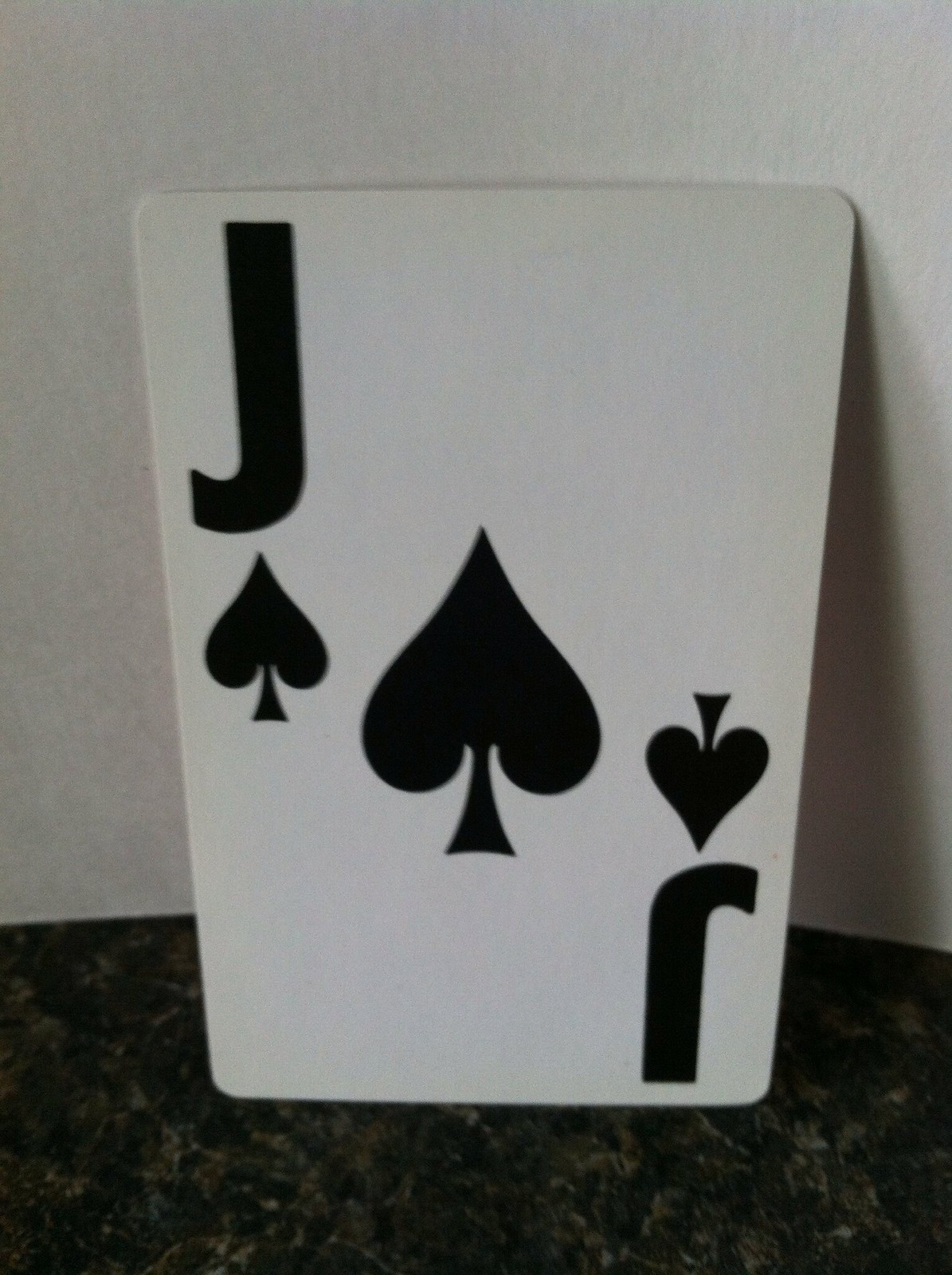The image depicts a Jack of Spades playing card standing upright against a textured white background. The card features a large black "J" in the top left corner, accompanied by a black spade symbol beneath it. Centrally, the card showcases the traditional Jack of Spades illustration. In the bottom right corner, there is an upside-down "J" with an inverted spade symbol placed above it. The card has slightly rounded corners and straight edges, adhering to the standard playing card shape.

The illumination in the scene suggests that the light source is positioned behind the camera and to the left, casting a shadow on the right side of the card. The white background, likely a sheet of paper, has a subtle texture. The surface upon which the card rests appears to be granite or a composite stone. This surface is predominantly black, interspersed with specks of brownish-gray and whitish-gray, contributing to its dark, intricate appearance.